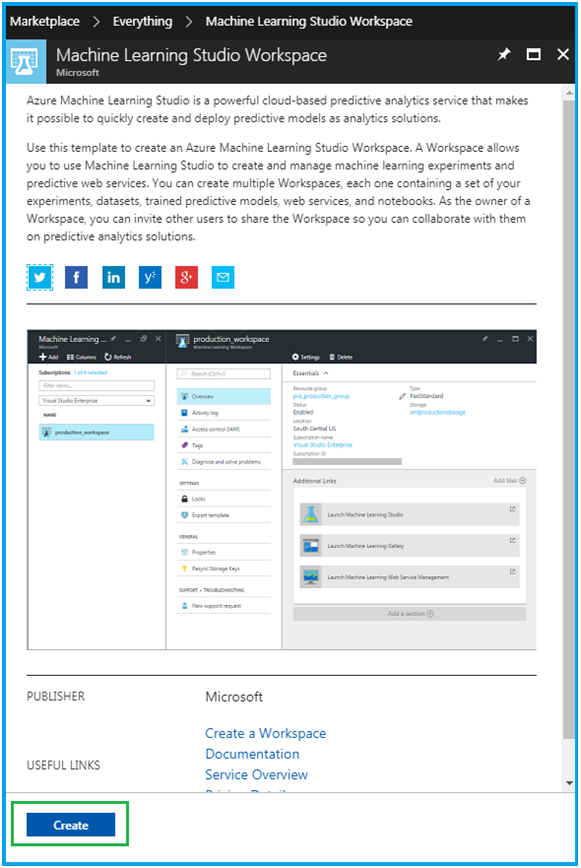The screenshot displays the interface for Microsoft's Azure Machine Learning Studio Workspace. The top left corner features the Marketplace icon, providing access to various services. Below it is the Machine Learning Studio Workspace section, highlighted by a blue graphic. The text adjacent to this graphic reads, "Machine Learning Studio Workspace, Microsoft."

There is a summary that outlines the features of Azure Machine Learning Studio: "Azure Machine Learning Studio is a powerful cloud-based predictive analytics service that makes it possible to quickly create and deploy predictive models and other solutions. Use this template to create an Azure Machine Learning Studio Workspace. Our workspace allows you to use Machine Learning Studio to create and manage machine learning experiments and predictive web services. You can create multiple workspaces, each one containing a set of your experiments, datasets, training, predictive models, web services, and notebooks. As an owner, you can invite other users to share the workspaces and collaborate with predictive analytics solutions."

On the right side of the screen, there are buttons for sharing on Twitter, Facebook, and LinkedIn. Additional icons likely represent Google services and email. Underneath, titles like "Machine Learning," "Production Workspace," and "Subscriptions" are visible, along with activity logs and access tags, presumably indicating user-specific logs.

At the bottom, "Publisher: Markzware" is noted alongside useful links like "Create a Workspace Documentation" and "Service Overview." To the right side, a blue button is framed by a green border, with an adjacent gray button providing further navigational options.